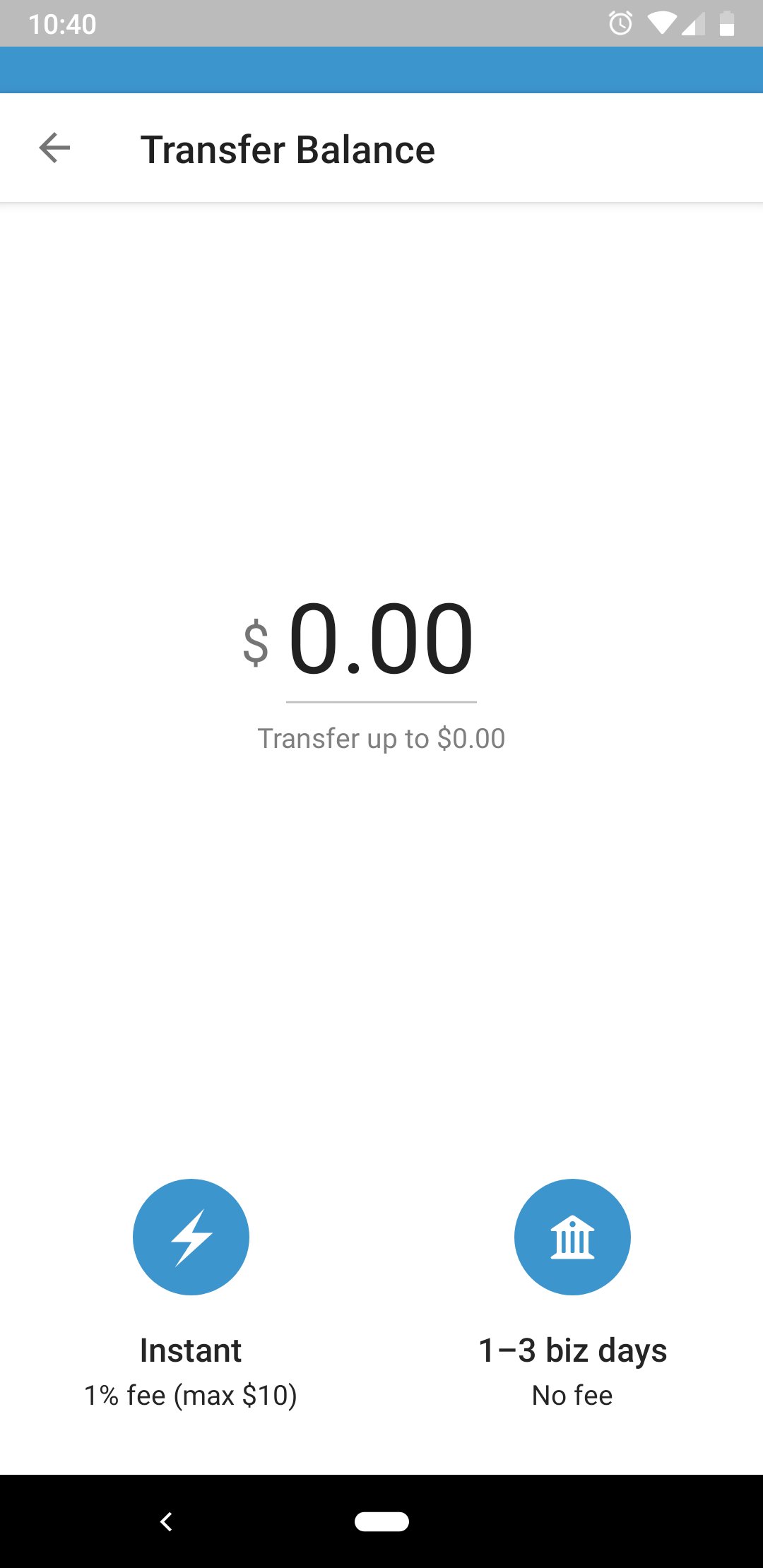The image captures a screenshot from a mobile phone's screen, which appears to be an interface for a financial transaction or money transfer application.

At the top of the screen, there's a gray strip featuring white icons. On the left side of this strip, the time is displayed as "10:40." On the right side, there are various status icons for alarm, Wi-Fi, mobile data, and a battery indicator showing it is half-full.

Below this gray strip, there's a blue strip with essential navigation elements. On the left side of the blue strip, there's a left arrow button, and beside it are the words "Transfer Balance." A thin gray line separates this section from the main transaction interface.

Centered prominently in the main interface, the text "0.00" is displayed, indicating the amount available for transfer. Below this, it states, "Transfer up to 0.00," with a dollar sign symbolizing the currency.

Further down, there are two blue circles with white icons. The left circle features a zigzag line inside and the word "Instant," followed by the text "1% fee, max $10" in parentheses. This indicates an immediate transfer option with a fee. The right circle contains an icon resembling a building or business structure and the text "1-3 Business Days, No Fee," indicating a standard transfer option without any fee.

At the bottom of the screen, there's a black band that includes a left caret (arrow) and a thick white line in the middle. While the interface closely resembles that of PayPal or another money transfer service, there are no explicit indicators confirming the exact application.

The primary colors used throughout the interface are gray, white, blue, and black.